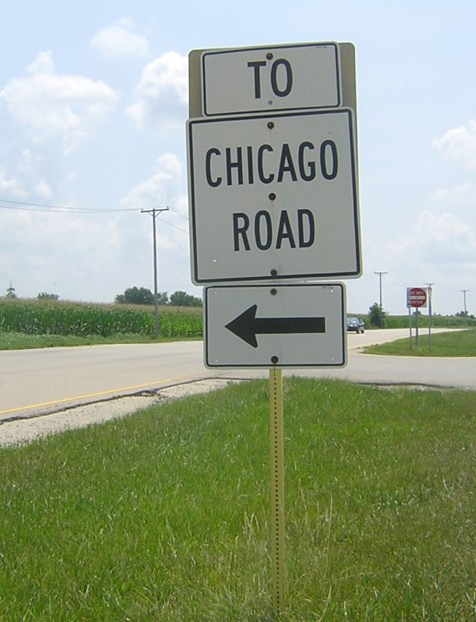The photograph, taken during the day, showcases a complex road sign situated in a grassy field beside a large, light gray highway. The road demonstrates signs of aging, with visible cracks and yellow stripes running along its length. The sign, composed of three separate white metal panels with black text and borders, is affixed to a yellow-tinted pole. The top panel reads "2TO," the middle panel says "Chicago Road," and the bottom panel features a black arrow pointing to the left. Surrounding the sign is light green grass, and further behind it lies a vast stretch of farmland with very tall corn stalks, their dark green leaves tipped with yellow.

On the left side of the image, an oncoming car can be seen traveling along the main road. Another road branches off to the right, creating an intersection. A "Do Not Enter" sign is visible in the field beyond the branching road. Power lines run parallel to the roadway, further emphasizing the rural setting. Above, the sky is light blue, adorned with wispy white clouds tinged with darker shades of blue at their bases. In the distance, a red stop sign with white lettering is also discernible, marking another point of interest on this expansive landscape.